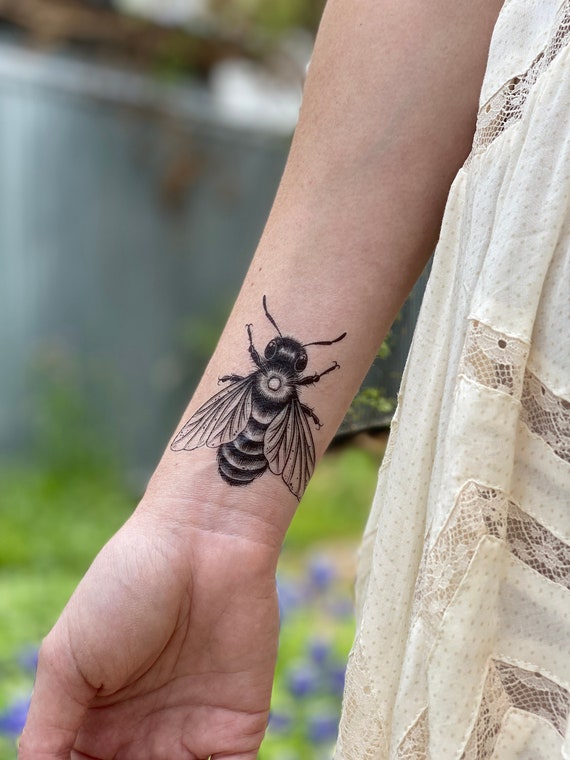The image depicts the inner lower arm of an individual with pale white skin, prominently displaying a large, detailed black and white tattoo of a bee. This intricate tattoo, situated just above the wrist and covering approximately one-third of the forearm, features distinct details such as the bee's head, eyes, antennae, legs, wings, and segmented abdomen characteristic of a bee. The individual is wearing a flowy, off-white cotton dress adorned with lace, and their arm is held down at their side. The photo is taken outdoors, with a blurred background suggesting a garden and a fence, giving the image a portrait-style feel.